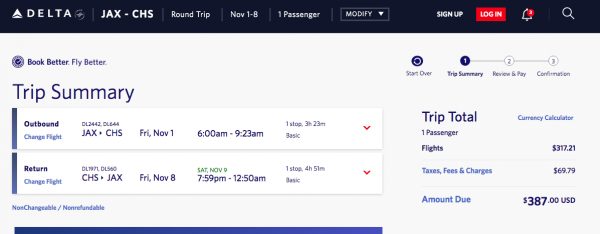A screenshot displays a digital Delta Airlines ticket. At the top, a black banner features the Delta logo alongside the airline's name. Below, the ticket information reads: "From JAX to CHS, Round Trip, November 1st through 8th, One Passenger." The interface includes a drop-down menu for modifications, as well as options to sign up or log in. A notification bell icon and a magnifying glass for search functionalities are also visible.

In a gray background with blue text, the phrase "Book Better, Fly Better" is prominently displayed. The screen allows several actions and provides a summary of the current trip. The trip summary section lists the outbound flight from Jacksonville (JAX) to Charleston (CHS) on Friday, November 1st, departing at 6 a.m. and arriving at 9:23 a.m. with a single layover lasting three hours.

The return flight is detailed below as departing from Charleston (CHS) to Jacksonville (JAX) on Friday, November 8th at 7:59 p.m. and arriving on Saturday at 12:50 a.m. This flight also includes one stop and a total duration of approximately four hours.

The total trip cost for one passenger is $317.21, with added taxes and fees amounting to $68.79, bringing the overall total to $387.00 USD.